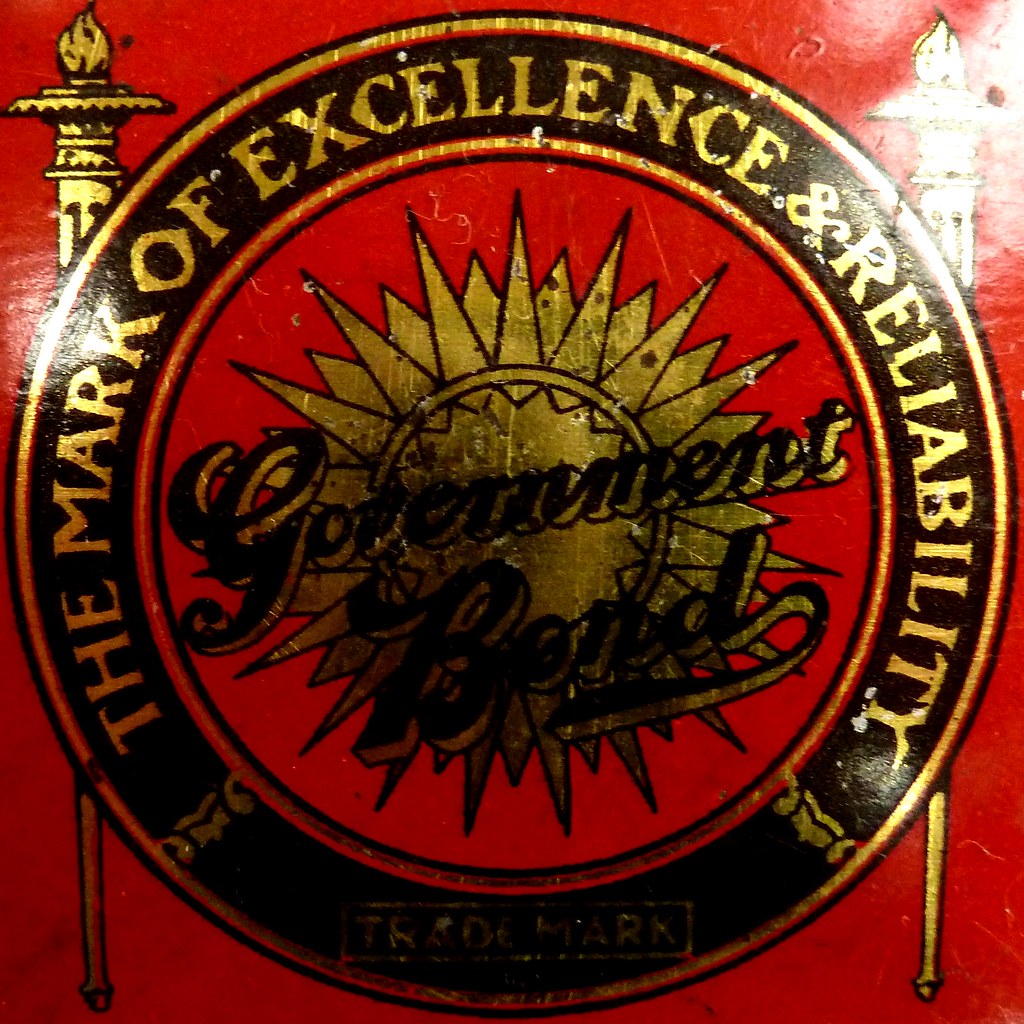In this large, square, solid red image, there is a noticeable textured background that appears to be painted on a metal surface. The image is very shiny, reflecting light prominently. At the center of this red background is a distinct circular label bordered with a gold and brown edge. The thicker outer brown border contains the words "The Mark of Excellence and Reliability" in gold lettering, curving from each side over the top to the other side. Below, at the bottom of this border, is the word "Trademark" enclosed in a thin gold rectangle, though it appears worn and slightly faded.

Within the circular label, the inner circle is predominantly red, featuring a gold sunburst design in its center. This sunburst is intricately outlined in black. Diagonally across the sunburst design are the words "Government Bonds" written in cursive, alternating in black and gold letters. The overall design gives the appearance of a label or logo, combining elements of gold, black, and red to convey a sense of prestige and reliability. On either side of the circular label, there are two large torch illustrations, adding to the intricate design.